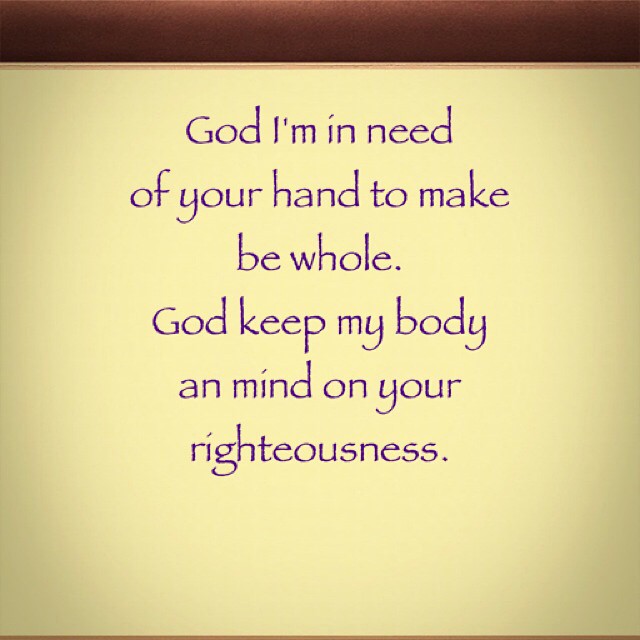The image is a digital design consisting of two sections. The larger bottom section, covering over 90% of the image, features a tan background with a gradient effect that is lighter in the center and darker around the edges. The top section is a thin brown rectangle, also with a gradient effect, creating a lighter center. The text is written in a deep purple, almost handwriting-like font, and reads: "God, I'm in need of your hand to make B whole. God, keep my body and A-N mind on your righteousness." The text contains two apparent typographical errors: "B whole" instead of "me whole" and "A-N" instead of "and mind." The design conveys an inspirational and motivational message, seemingly put together quickly, yet remains simple and minimalist. Only the initial "G" in "God" is capitalized in both sentences.